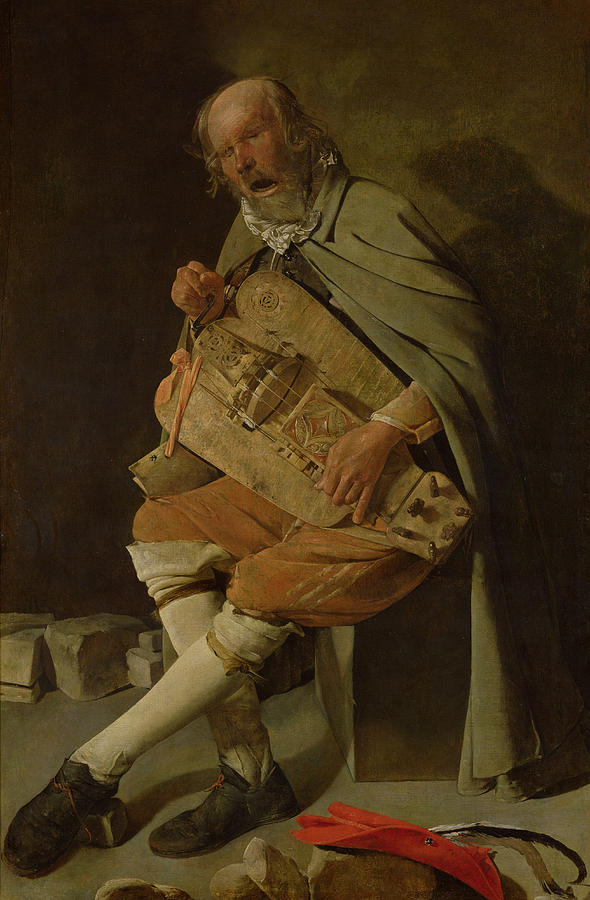The painting depicts an elderly man, likely in his 80s, with gray, scraggly hair, bald on top, and a white beard. He is seated, possibly on a wooden block, and is dressed predominantly in brown attire, including a cloak that covers his shoulders and extends down to the floor. He also wears knee-length pants that tuck in at the knees, white knee-high socks, and brown shoes. The background is a muted greenish-brown.

In the painting, the man is engaged with a medieval musical instrument, possibly a lute or a lyre, which he holds in his hands. His left hand is on the strings, and his mouth is open as if he is singing. He is wearing a gold-colored shirt under his cloak, and a red glove can be seen on the floor to the right side of the painting.

Beside him, there appears to be a table with what looks like loaves of bread on it, covered partially by a white or red serving cloth. The setting suggests a mix of agony and passion, captured in the man's expressive, open mouth as he strums the instrument.